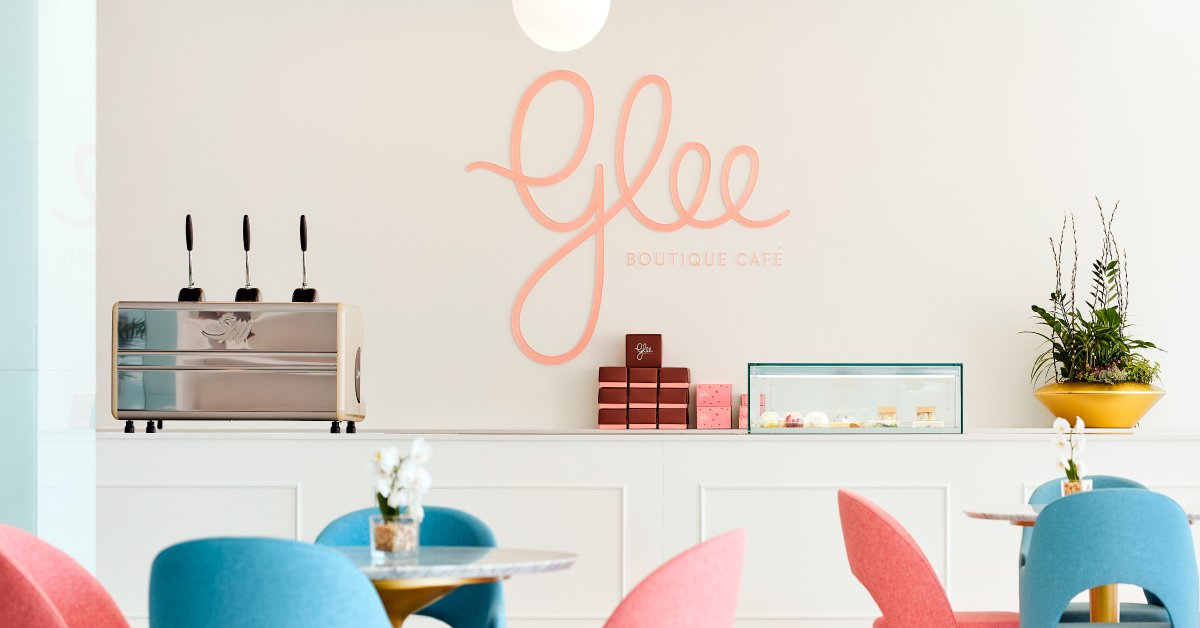This brightly lit photograph captures the inviting interior of Glee Boutique Cafe. Dominating the white wall in the center of the image, the word "GLEE" is written in a peachy-pink cursive, with "Boutique Cafe" in smaller capital letters directly below the last 'E'. To the left of this sign sits a rectangular tan container approximately two feet high, partially obscured by a stack of Glee-embroidered boxes—ten in total—with the top box showcasing the cursive branding. These boxes, featuring pink bases and red lids, are positioned next to two additional pink boxes adorned with red dots and several smaller matching boxes. Adjacent to this display, a glass case presents domes and miniature house sculptures. On the rightmost side of the counter under the Glee sign, a brass-potted plant adds a touch of greenery. 

Further down, the seating area features two round glass-top tables. Each table is elegantly decorated with a white flower centerpiece in a glass vase. Around these tables are a mix of colored chairs—two blue and one pink at the nearest table, and two blue and two pink at the farther table. The leftmost wall of this inviting cafe is painted in a calming cyan blue, complementing the overall bright and cheerful ambiance.